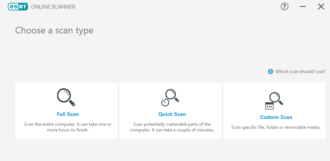The image shows a somewhat blurry screenshot of an online virus scanner interface. In the upper left-hand corner, the header reads "Online Scanner," accompanied by a white and green oval logo, though the text within the logo is illegible. Below the header, there is an option to "Choose Scan Type" surrounded by a light gray background. 

Three horizontally aligned white cards represent the scan options, each featuring a magnifying glass icon:
1. **Full Scan**: A magnifying glass icon suggesting a comprehensive check.
2. **Quick Scan**: A magnifying glass combined with a clock, indicating a rapid inspection.
3. **Custom Scan**: A magnifying glass paired with an entry form icon, allowing personalized scan settings.

While there are detailed descriptions of each scan type beneath the icons, these details are too small and faint to be discerned from the image. 

In the upper right-hand corner of the screenshot, three additional icons are depicted:
- A question mark inside a circle, presumably representing a help or support feature.
- A straight line dash, indicating the option to minimize the application.
- An 'X,' which allows the user to close the application.